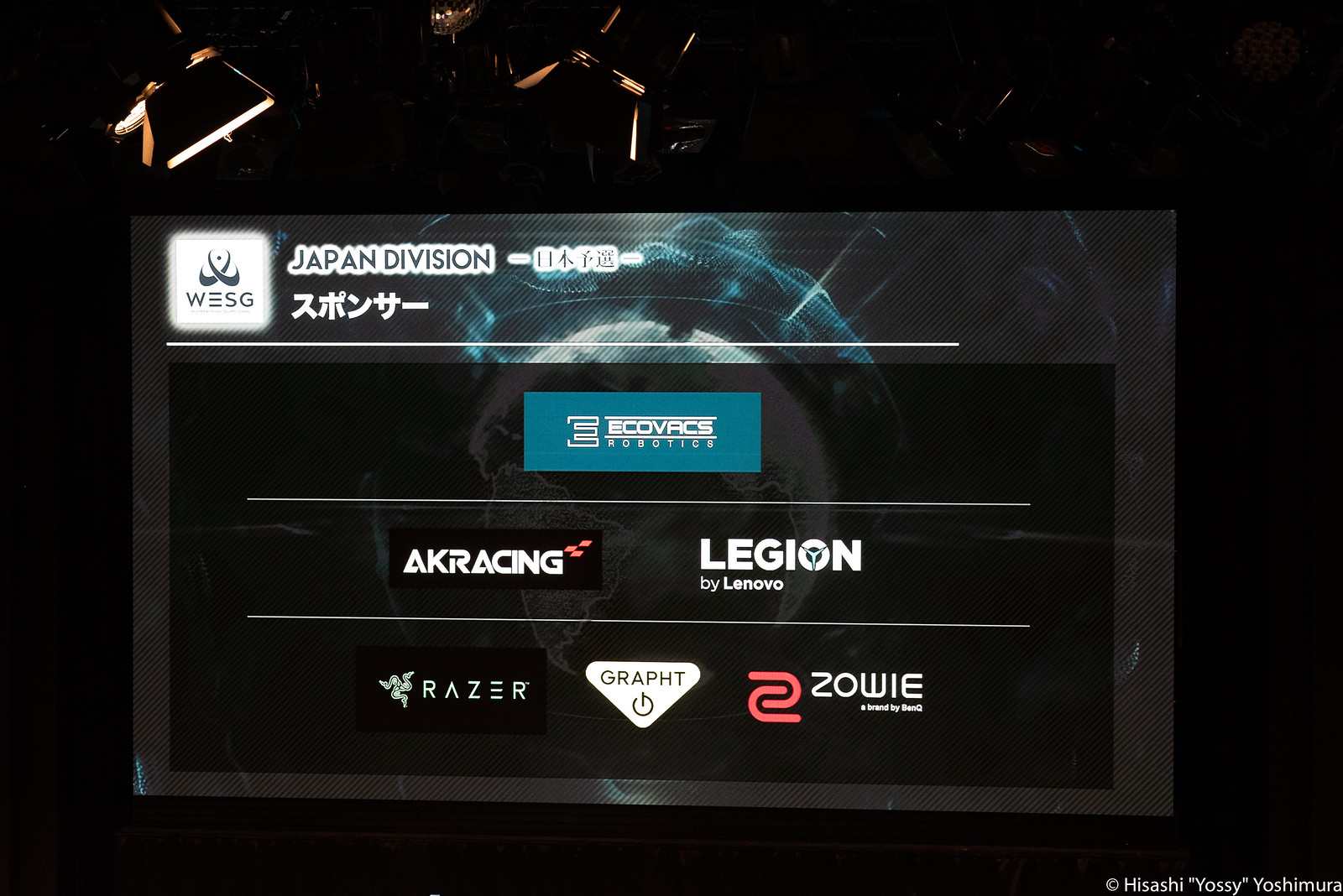The image appears to be a digital projection or screen display, possibly from an esports competition or event. The background is entirely black, creating a stark contrast with the other elements. At the top, there are floodlights or spotlights, though they are pointed away, only allowing some light to illuminate the projection from the flaps that obscure them.

Centered on the screen is the logo for WESG, which resembles two Nike swooshes on their sides with a dot in the middle. Below this, "Japan division" is prominently displayed with Japanese characters adjacent, likely translating the text. This text is highlighted with a white outer glow, making it stand out against the background.

Further down, a series of brand logos are arranged, suggesting sponsorship or endorsement alignments for the event. These include:
- Ecovacs Robotics within a teal rectangle, marked with an 'E'
- AK Racing displayed in a black block with a small red checkered flag
- Legion by Lenovo 
- Razer, identified by its distinctive green font and snake logo
- Graft
- Zowie, denoted by its stylized red 'Z'

Each of these logos retains its unique brand design. The bottom right corner of the image contains a faint watermark. Altogether, the setup and branding indicate a structured and professional presentation, likely connected to a video game competition or an esports tournament.